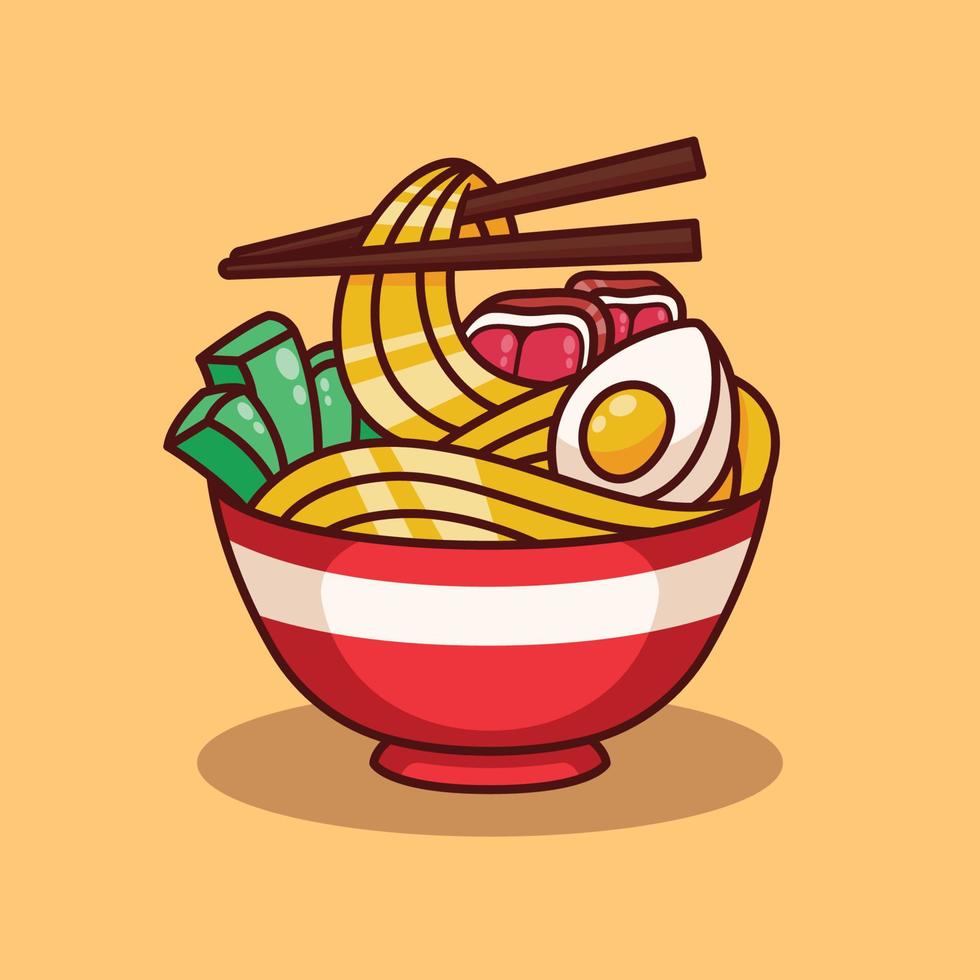The image showcases an animated, cartoon-styled drawing of a bowl of ramen centered against a light tan-yellow background, with plenty of shading beneath the bowl. The ramen is served in a red bowl, featuring a white stripe horizontally across it. The contents of the bowl include a prominently displayed halved egg, revealing both the yolk and egg white, with noodles artistically looped upwards, resembling ice cream. To the left within the bowl, green bamboo shoots can be seen. At the very top, there's an illustration of red meat, likely representing some sort of cut meat. Intertwined with the noodles are brown chopsticks, adding to the detailed depiction of the dish. The drawing is vibrant and detailed, making the scene bright and clearly visible.